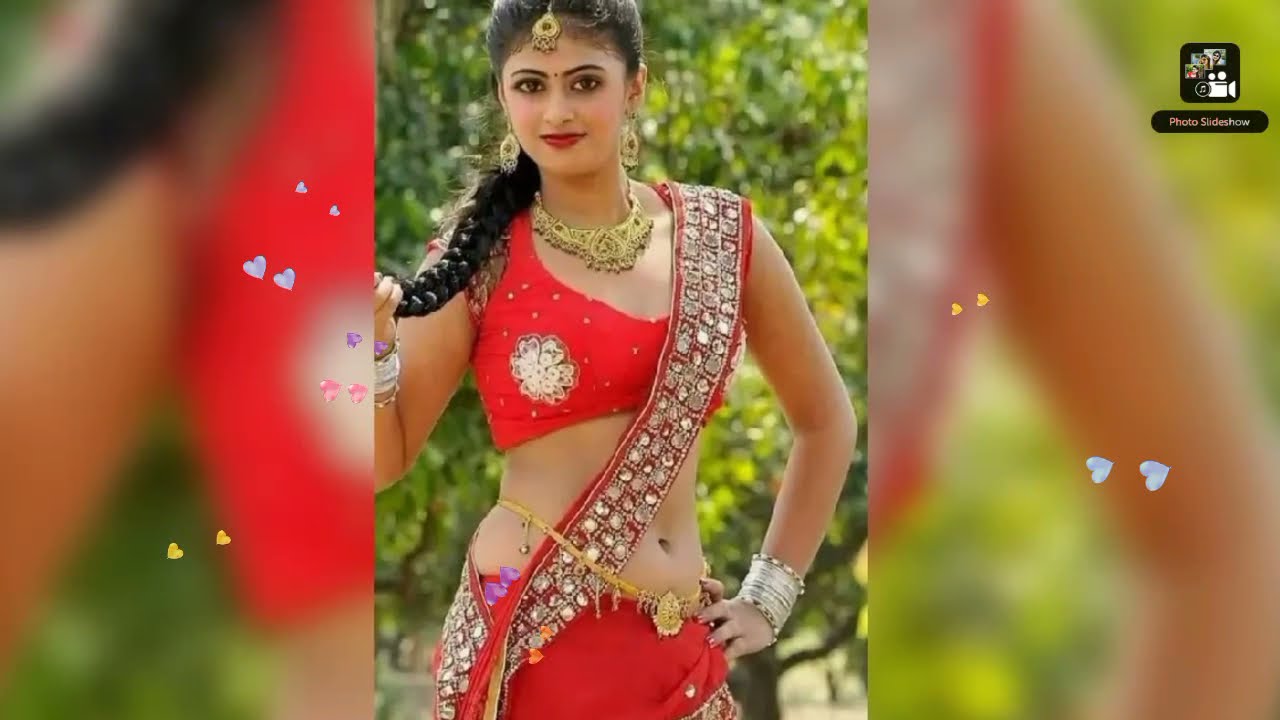This is a vibrant color photograph featuring a young woman of Indian descent, elegantly dressed in traditional dance attire. The composition of the image is wide and rectangular, with a sharp, clear central portrait flanked by blurry, enlarged close-ups of the same image on the left and right. These side panels are sprinkled with multicolored hearts in shades of blue, yellow, pink, and purple. 

The central figure stands confidently against a backdrop of verdant green foliage, likely a bush. She is adorned in a striking red ensemble, comprising a short top, a flowing skirt, and a shawl richly embellished with silver jewels. Her light brown skin and expressive dark eye makeup highlight her captivating presence. She accessorizes with an ornate gold necklace that matches her large gold earrings, and a delicate gold chain cinches her midriff. Additionally, she sports silver bangles on both wrists, a medallion headpiece, and a gold belt with a medallion accent over her left hip. 

Her long dark hair is styled into a braided ponytail, which rests over her right shoulder and is held delicately in her right hand. She wears a subtle, half smile, adding a touch of warmth and allure to her poised stance. This richly detailed photograph captures both the elegance of traditional Indian attire and the serene beauty of its wearer.